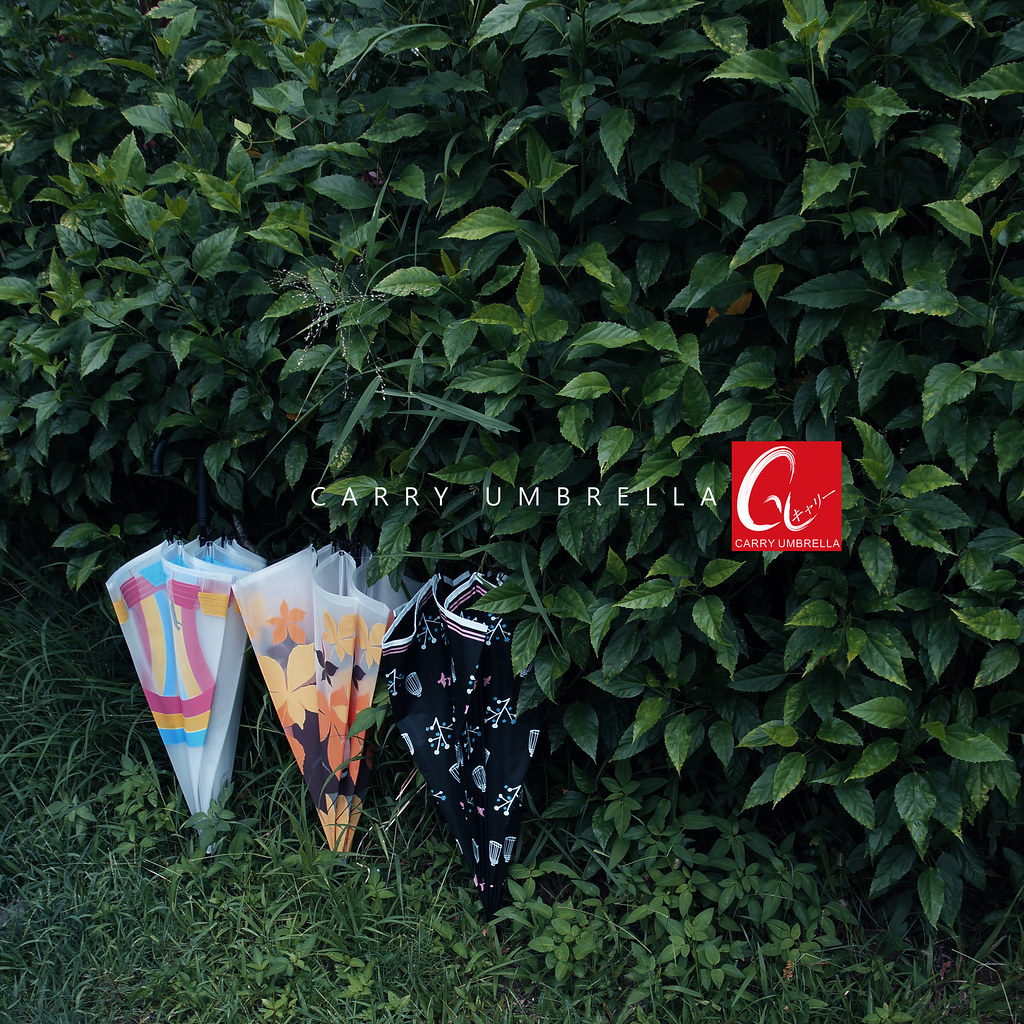This promotional photograph from an umbrella company features a dense backdrop of leafy green foliage, transitioning into wild grass with the occasional weed at the bottom of the image. Centered prominently are three upside-down, nearly closed umbrellas resting against the shrubbery. 

The umbrella on the far left is a translucent white with soft pastel stripes in blue, yellow, and pink, and has a black handle. The middle umbrella is also translucent white, adorned with an orange, yellow, and black floral pattern, accompanied by a black handle. The rightmost umbrella is predominantly black, decorated with intricate white designs, possibly resembling star constellations or branches, complemented with a white border at the top.

In the middle of the photograph, white text reads "Cary Umbrella," immediately next to a red square logo featuring a stylized, large white "C" and a smaller "U," with the words "Cary Umbrella" also inscribed within the logo.